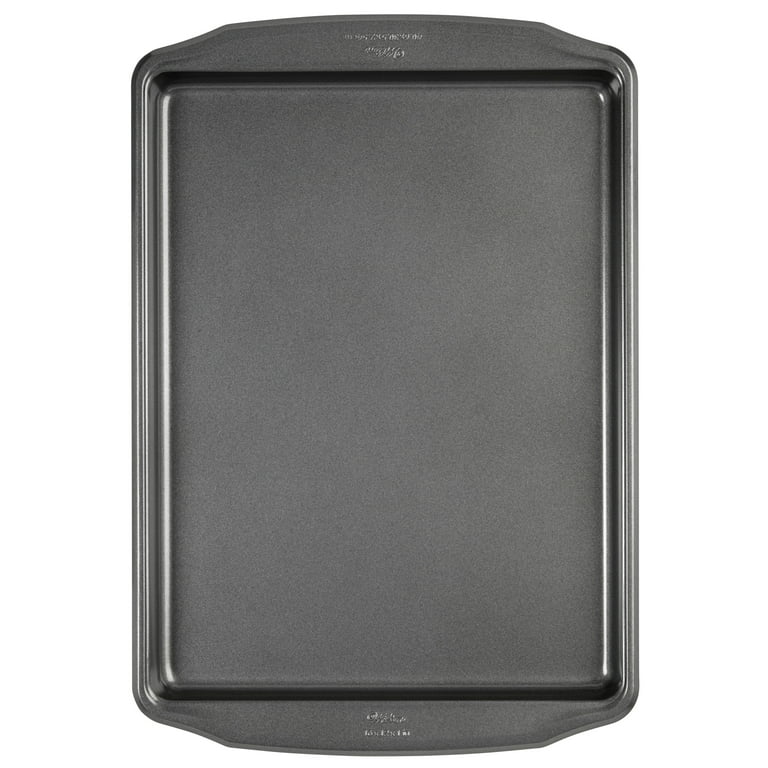This image depicts a medium to large, brand-new cookie sheet or baking pan, commonly found in households. The sheet, likely made of non-stick aluminum, features a smooth, dark gray surface that's devoid of any scratches, indicating it has never been used. The cookie sheet has a rectangular baking area with slightly curved edges at the top and bottom, and it is designed as a single, seamless piece with integrated handles for easy maneuvering. The manufacturer's name is stamped along both the top and bottom edges, though it is not legible. Positioned flat against a white or neutral background, the top-down view suggests that the image might be used for advertising purposes. This versatile and slim baking sheet is perfect for making an array of baked goods, from cookies to chicken, and its sleek design would fit easily into a kitchen drawer.